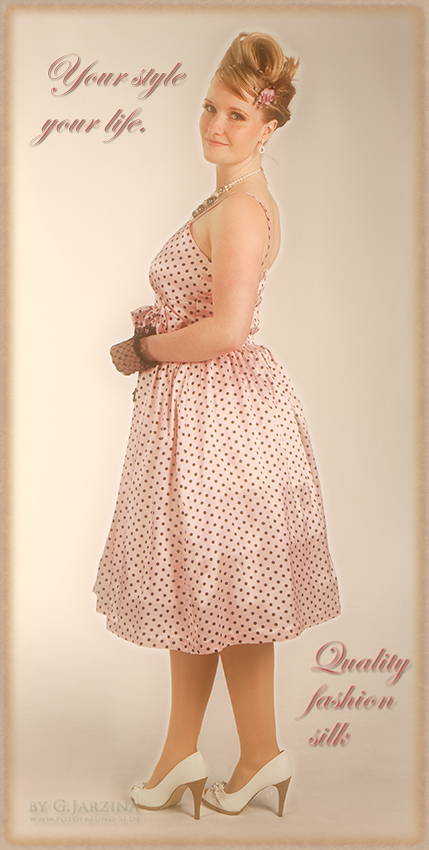The image features a Caucasian model in a retro, 1950s-style ensemble. She is adorned in a calf-length, satiny pink dress with small black polka dots, which has a tight bodice and a slightly poofy skirt held up by spaghetti straps. Her hair, blonde and elegantly arranged in a curled updo, is accented with a pink floral clip. She is striking a pose in profile but gazes directly at the camera over her left shoulder. Her accessories include black lace gloves, a diamond and black necklace, and matching earrings. She completes her look with white high heels featuring tan heels. The backdrop of the image is a creamy white, framed with a tan border that complements the model's attire. Prominently displayed in the upper left corner, the script text reads, "Your Style, Your Life," while the bottom of the image contains the phrase "Quality Fashion Silk" in the same script font. Additionally, a subtle watermark in the bottom left corner identifies the artist or designer as G. Jarzina.